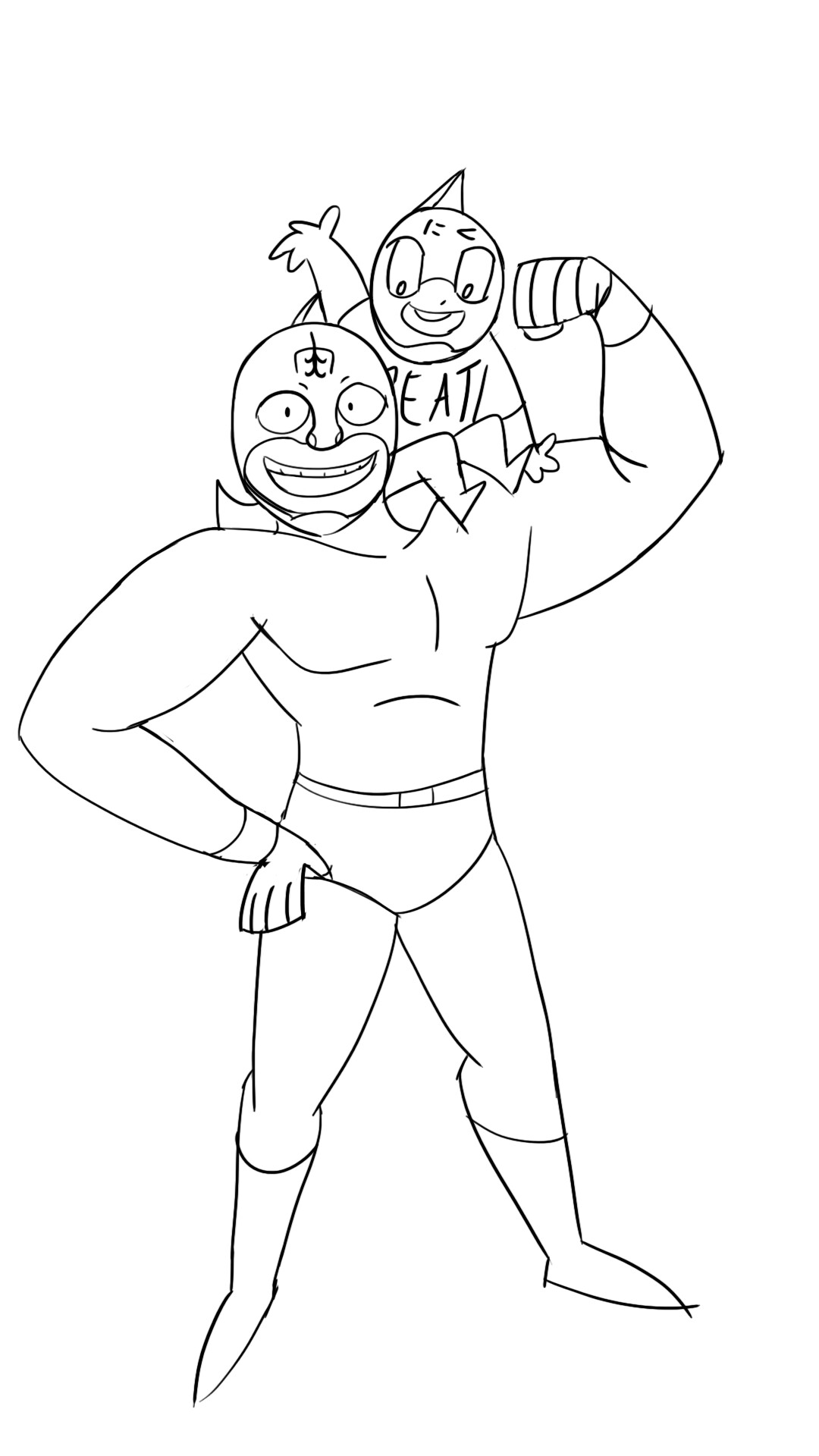This black-and-white line drawing, likely from an anime or manga due to the proportions and style, features a muscular superhero character posed confidently. The character stands with his feet apart, right arm on his hip, and left arm flexed, showcasing his muscles. He wears boots, trunks, and a belt reminiscent of a luchador or classic superhero costume. Notable details include a mask, a large, well-defined mouth, and a bald head. Perched on his shoulder is a small, masked child-like figure with a shirt that reads "EAT." The image has a clean, simple line work style with uniform thin line weights, set against a white background.